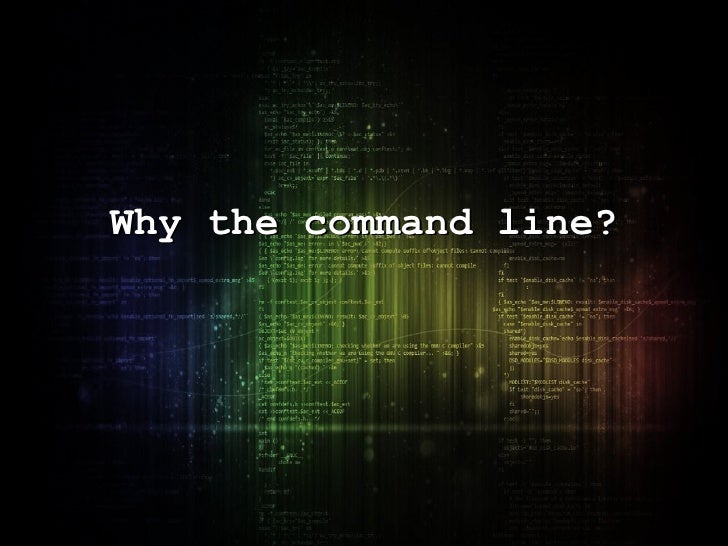This is a detailed color image that presents a square media piece with completely black edges for dramatic effect. The central focus is a white, typewriter-style text that questions, "Why the command line?" This text, capitalized for emphasis at the start of "Why," is positioned slightly above the center of the image, set against a stylized depiction of several computer screens. These screens display rows of computer code, too small and blurred to decipher, with streaks running vertically across them. The coding screens exhibit a gradient transition of colors: blue on the left, shifting through green and yellow, and culminates in red on the right. The image composition maintains a high contrast as it darkens towards the borders, especially in the corners, compelling the viewer's attention towards the illuminated, central text and the underlying coding patterns.